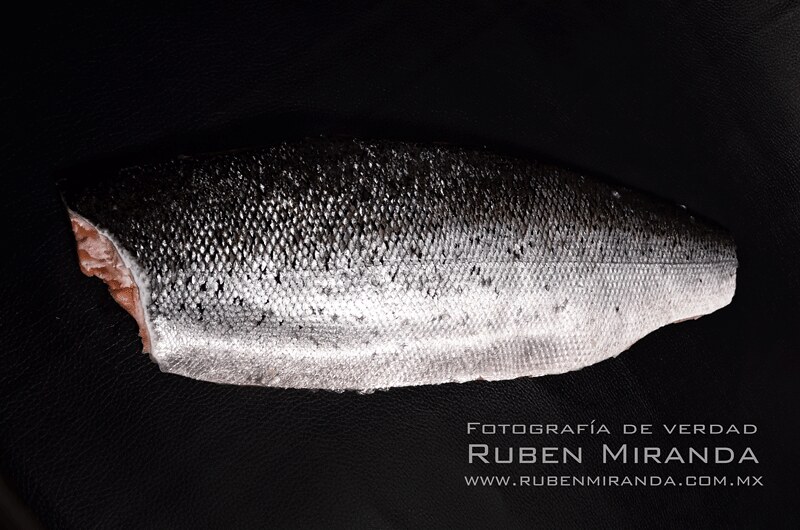The image features a fish fillet set against a deep black background. The fillet, captured in the center of the frame, is a mid-section cut with both its head and tail removed, showcasing the textured scales and flesh. The upper part of the fillet is adorned with dark, silvery-black scales peppered with small black specks, while the lower part gleams brilliantly under light, presenting a nearly white, silvery sheen. A hint of the salmon's characteristic peach-pink flesh is visible along the left edge of the fish. The cut edges appear slightly jagged. Positioned in the lower right corner of the image is the phrase "Fotografia de Verdad" in small letters, followed by the photographer's name, Ruben Miranda, and his website, www.rubenmiranda.com.mx, indicating that the photograph likely originates from Mexico. This detailed image, ready for culinary preparation, beautifully contrasts the dark and light elements of the fish's scales, creating a visually captivating piece.